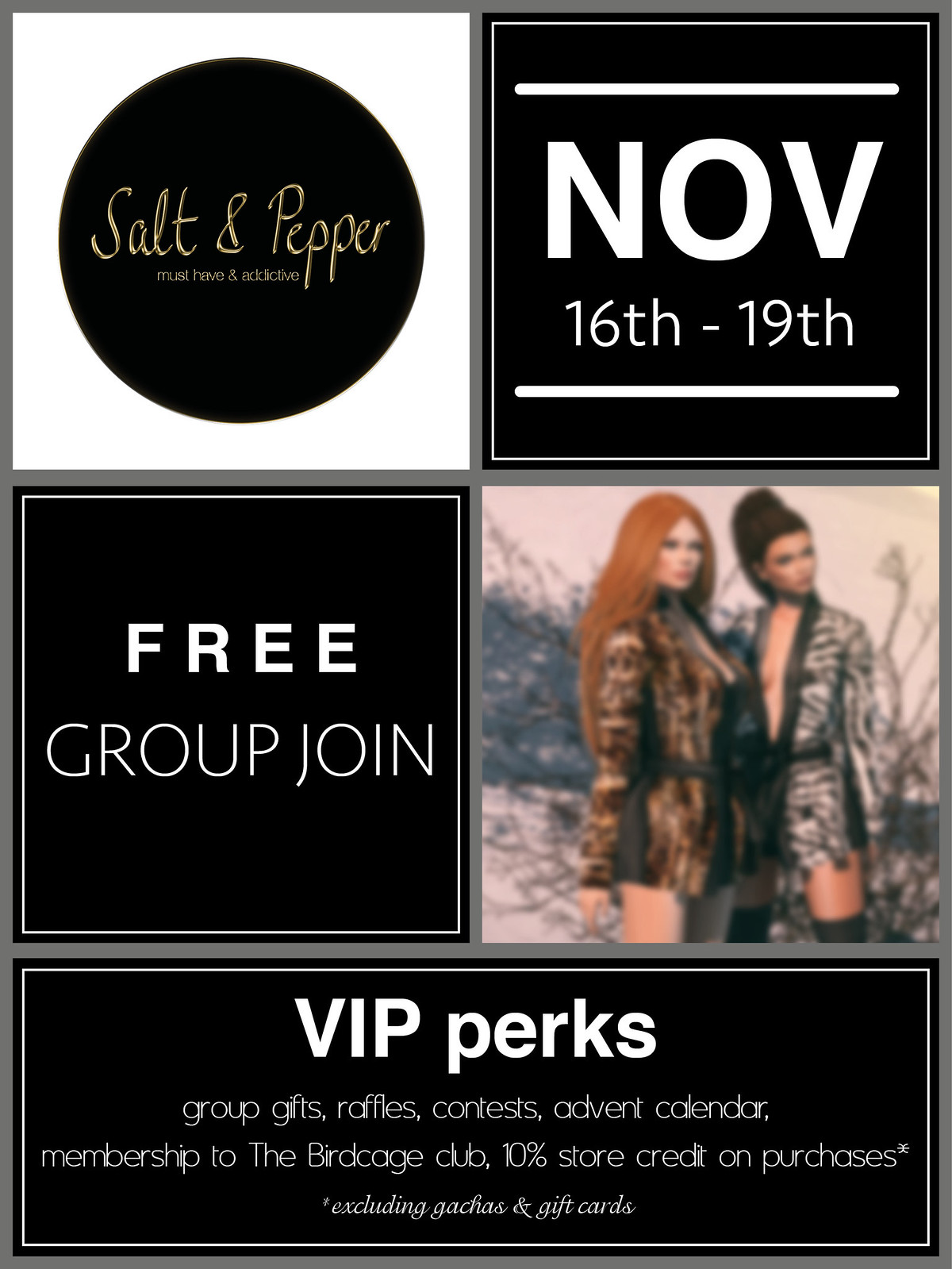This image is an advertisement for Salt-N-Pepper, segmented into a collage of five distinct sections against a white background. The upper left features the logo – a black circle with golden lettering reading "Salt-N-Pepper: Must Have and Addictive." Beside it, in a separate black square with large white letters, are the dates "November 16th - 19th." Below the logo, another square declares "Free Group Join" in bold white text on a black background. Adjacent to this is an image of two women resembling AI-generated or 3D avatars, one with long orange hair and the other with dark, pulled-back hair, both appearing in sensual attire. The bottom footer, a black rectangle, lists extensive VIP perks in white text: "Group Gifts, Raffles, Contests, Advent Calendar, Membership to the Birdcage Club, and 10% Store Credit on Purchases," noting the exclusion of gachas and gift cards. The cohesive design and enticing offers emphasize the benefits of joining the group for free.